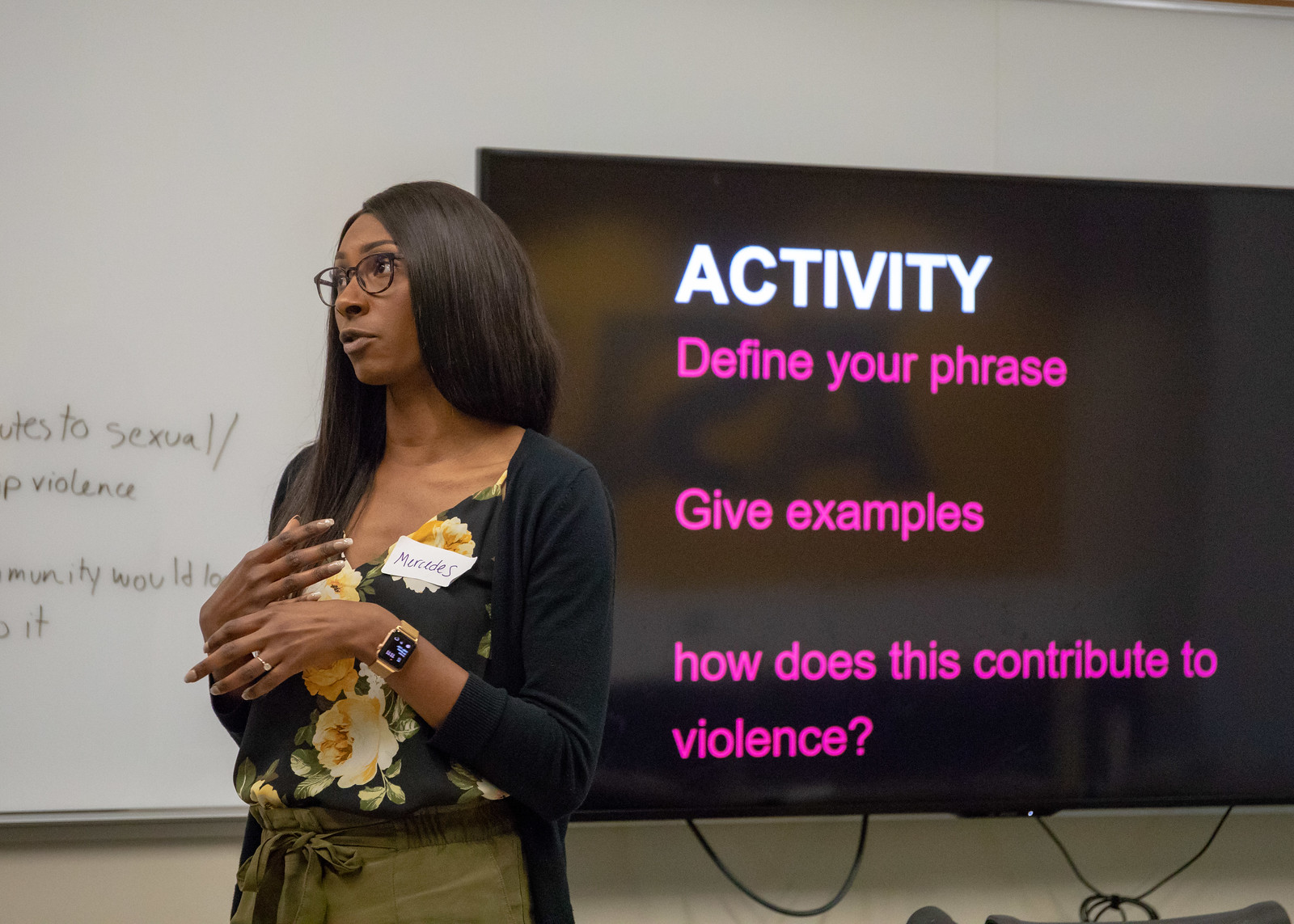In the image, a black woman with long black hair and eyeglasses stands at the head of a classroom, seemingly engaged in delivering a lecture. She is wearing a floral-colored shirt paired with a black sweater, and a gold Apple watch adorns her wrist. A name tag on her chest reads "Mercedes." She appears to be addressing an audience or a class, with a large whiteboard visible behind her. The whiteboard has some written content, though the legible parts include phrases like "sexual violence" and "community wood." To her right, a large screen or TV displays text related to her lecture. The screen features the word "Activity" in large white letters at the top, followed by three magenta-colored bullet points: "Define your phrase," "Give examples," and "How does this contribute to violence?" The backdrop of the scene is a black background with yellow flowers, adding to the detailed setting of the educational environment.